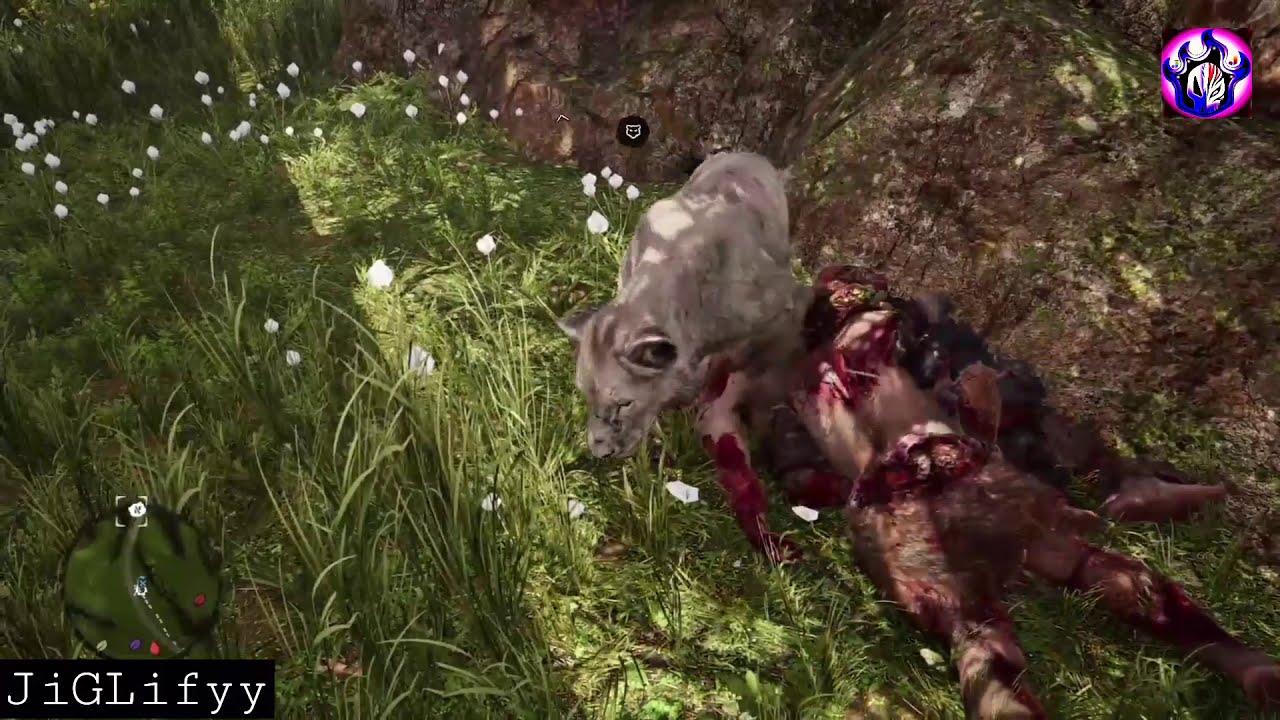This image appears to be a blurry, computer-generated screenshot, likely from a video game or an animation. The scene is set in a grassy and rocky pasture with some white flowers scattered around. Centrally, a severely injured or possibly dead man lies on the ground, his body showing significant wounds and blood, suggesting the possibility that he might even resemble a zombie due to his visibly torn and battered condition.

Standing nearby, there is a large, grayish animal, which is difficult to identify clearly due to the blurriness of the image; it could be a bull, cow, or more probably a panther or a large cat, given the context of blood and possible predation. This animal appears to be either inspecting or guarding the bodies, adding a menacing atmosphere to the scene.

In the top right corner of the image, there is a distinct emblem featuring a skull enveloped in blue flames, contributing to the overall dark and ominous tone. At the bottom left, a black box contains the text "Jigliffy" in white lettering, which could be the name of the game or a signature watermark.